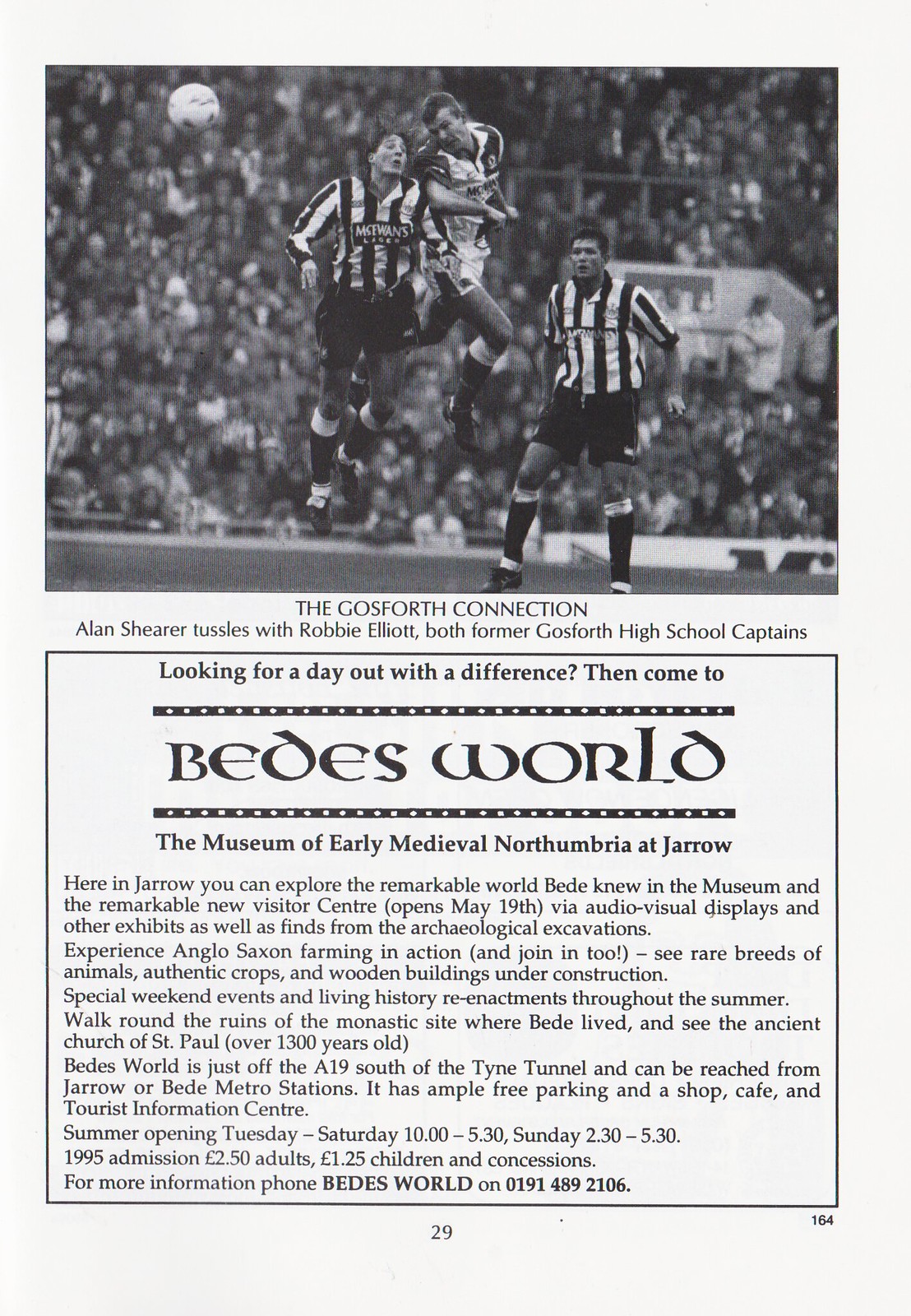The black and white image on page 29 of an old sports magazine features what appears to be a soccer match. In the scene, three figures are prominent: two of them, dressed in black and white striped shirts and black shorts, suggesting they might be referees, though their actual role could be as players, are caught mid-air in an attempt to head the ball. One of these striped-shirt figures is airborne next to a player in a white soccer outfit who also appears to be heading the ball, with the ball visible in the top left of the image. Another figure in a striped shirt stands flat on the ground, and behind them, a large, blurred crowd fills the stands. 

Beneath the photo, there is a caption, "The Gosforth Connection. Alan Shearer tussles with Robbie Elliott, both former Gosforth High School captains." Further down, an advertisement invites readers to "Bede's World, the Museum of Early Medieval Northumbria at Jarrow." The detailed text explains that Bede's World offers insights into Anglo-Saxon farming, rare breeds of animals, and historical reenactments, with ample facilities and various operational hours. The ad additionally provides contact information for visitor inquiries.